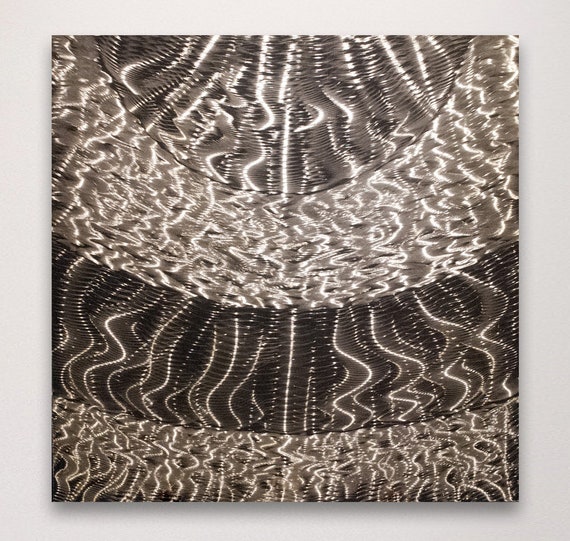The image features a central abstract design set against a white background. Dominating the scene are intricately patterned areas of dark grey and black, adorned with dotted and thick, serrated white lines that create a visually dynamic composition. The texture and layout evoke impressions of lace or a circus tent, with a notable band in the middle that appears circular and silvery, adding a shiny, reflective quality to the ensemble. Vertical elements within the design resemble tightly grouped gold springs, both loose and flattened, creating a dual-ringed structure that encompasses the central features. These elements, combined with horizontal wavy lines curving into half-circle shapes and streaks of white light, give the image a reflective, almost hall-of-mirrors effect, with light seeming to bounce and shimmer throughout the intricate, abstract arrangement.